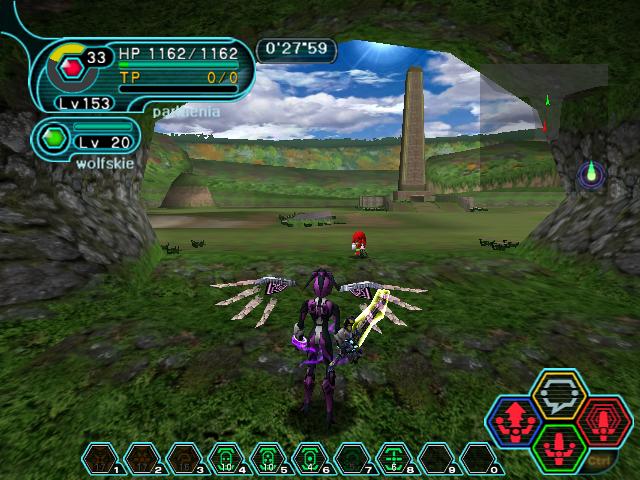This detailed screenshot from an early 2000s-style video game showcases a vibrant outdoor scene with lush green grass and scattered gray rocks under a blue sky with the sun peeking through fluffy clouds. Dominating the forefront is a relatively tall purple character adorned with white wings and wielding a large sword. This character stands out in the middle of the screen, facing a vast, green meadow. In the distance, there is a small red character that resembles Knuckles from Sonic, adding an element of familiarity. Behind this red character, a tall, gray stone tower rises prominently. The game's heads-up display is rich with information; the upper left corner shows stats like TP 0/0 and various numbers, while the bottom section is filled with pendants and colored lights symbolizing different game elements. Notably, one of the names listed is 'Wolfski' at level 20, suggesting it may be a party member, while the main character appears to be at a higher level, specifically level 153.